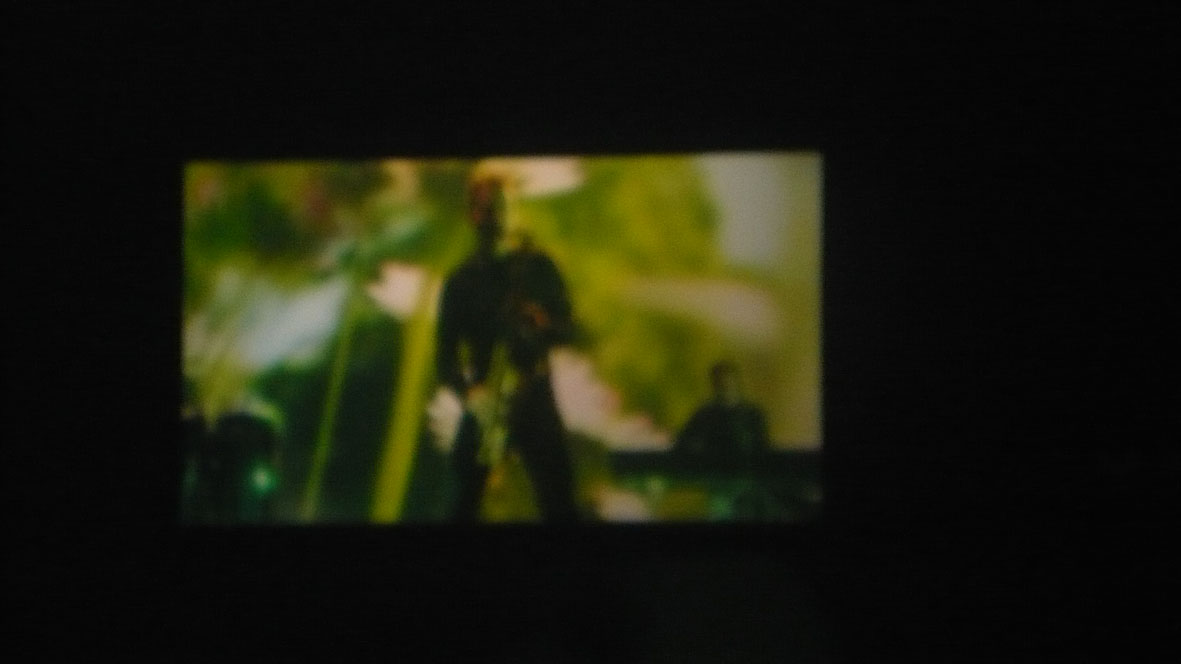In this blurry image, we observe a scene that appears to be a band performing, possibly displayed on a television or a large screen such as at a concert or movie theater. The image features a dark black horizontal rectangle with a central rectangular display showing the performance. The lead singer, situated towards the left, is playing a guitar or saxophone and is dressed in a dark black long-sleeve shirt and pants. Next to him on the right, a band member plays a keyboard, identifiable by its long, black rectangular shape. In the background, there are swirly lights in shades of light and dark green and white, suggesting an outdoor setting or a well-lit stage with a greenery backdrop. The scene is further complicated by hints of a possible drum set on the left side, though it's obscured and difficult to confirm due to the image's overall blurriness.